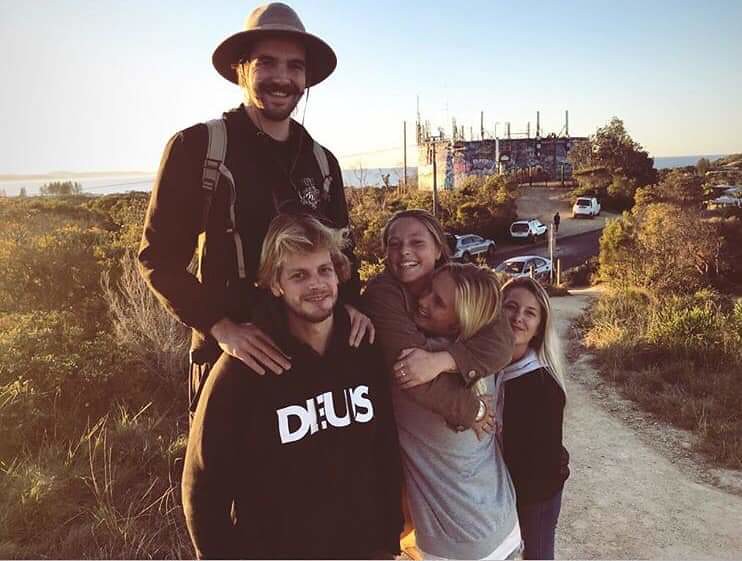This photograph captures a group of five Caucasian individuals, likely a family or close friends, standing on a dirt road amidst a rugged, hilly terrain with sagebrush and grasses in shades of khaki green, grey, and pale brown. The backdrop features a partially constructed house and a row of parked Volvo station wagons and other cars. In the distance, the horizon suggests a seashore, enhancing the scenic coastal vibe.

The group consists of two men and three women, all smiling broadly. One man, possibly in his 30s, stands behind the group with his hands gently placed on the shoulders of a younger man. This older man is identifiable by his fisherman's hat and small backpack, which might indicate he's standing on a rock to appear taller. The younger man, with streaky blonde hair, wears a noticeable black hooded sweatshirt emblazoned with the white text "DEUS". 

The three women, all blonde, exhibit youthful features, likely in their late teens or early 20s. Two women hug each other warmly, one with her back to the camera. Another woman's face peeks out from the side, smiling directly at the camera. The lighting, potentially from a sunrise, bathes the entire scene in a soft, warm glow, contributing to the overall cheerful and intimate ambiance of this outdoor snapshot.